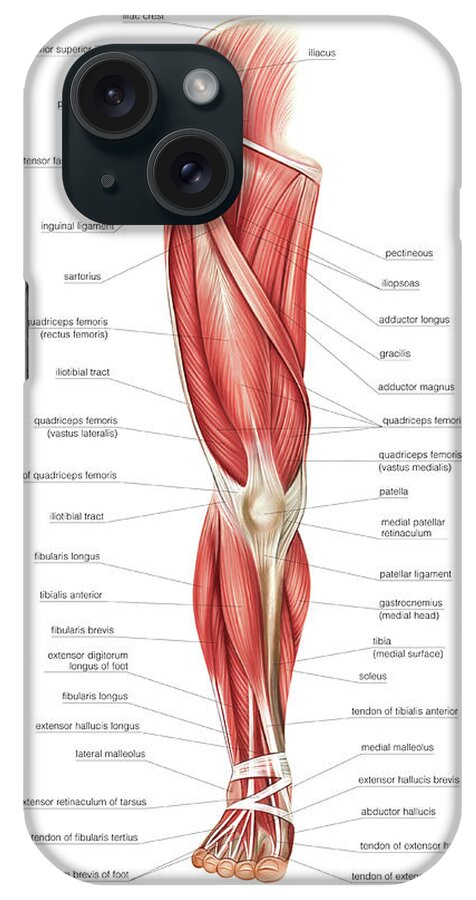The image shows the back of a cell phone, possibly an iPhone, displaying a highly detailed anatomical diagram of a human leg. The diagram spans from the hip area to the toes and reveals the internal structure, including bones, muscles, and tendons. The leg is prominently featured in the center with a white background, allowing the red muscles and white tendons to be clearly visible. Both sides of the leg are labeled with Latin medical terminologies, such as "quadriceps," "tract," "longus," "pectineus," "agranius," and "gracilis," each term underlined in black lowercase letters. Lines connect these labels to their corresponding parts on the diagram. The phone case also includes a camera in the top left corner, featuring multiple lenses.